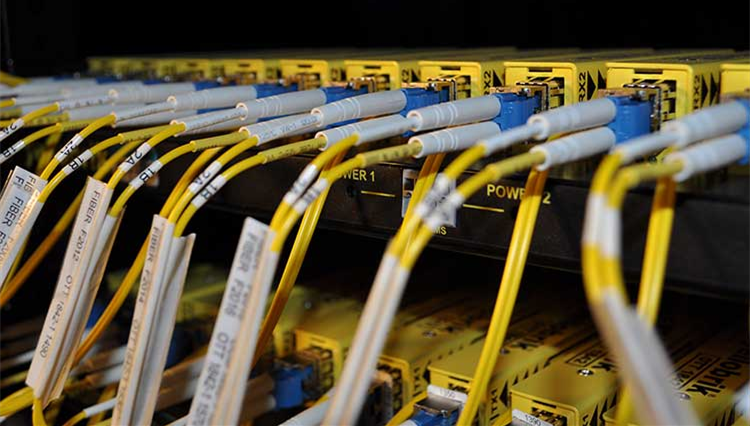This is a detailed landscape photograph of a server or power rack setup with a black background. The image shows two rows of identical yellow box-shaped devices, potentially power units or networking hardware, labeled with "Power 1" and "Power 2". Each yellow box features black writing and symbols. From each box, two sets of cables emerge. These cables have a consistent color pattern: initially white, transitioning to yellow. Each cable connects to the yellow box through a blue connector and is organized by labels indicating their function and position, such as "1B" and "2A". The cables appear to be labeled "fiber" and bear serial numbers. The setup is meticulous, with cables evenly spaced and precisely labeled, indicating a highly organized and possibly industrial or data center environment. The labels and structured arrangement suggest a focus on clear identification and management of connections, possibly for internet or networking purposes.